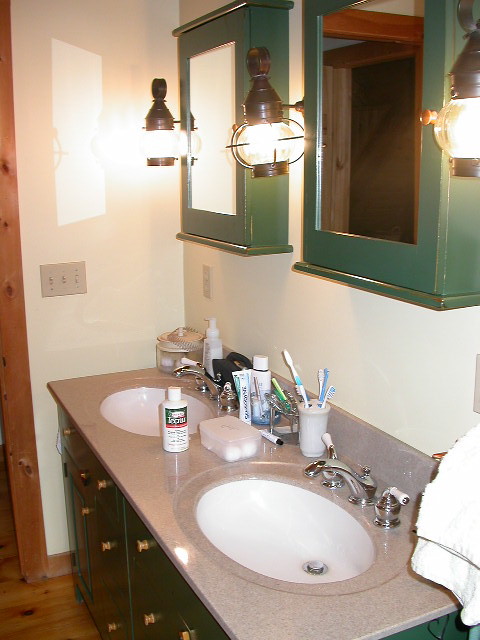This detailed image captures a double sink vanity in a well-appointed bathroom. The vanity showcases a luxurious stone or marble countertop, featuring two pristine white sink basins. Each sink is fitted with an elegant silver faucet, complete with two handles that feature white plastic grips for easy operation.

The countertop is adorned with an array of personal care items pressed neatly against the back wall. Among these are at least five toothbrushes stored in a holder, a tube of toothpaste standing upright, a glass jar filled with cotton balls, and various other tubes and bottles.

Above each sink hangs a green-framed mirror, approximately a foot and a half above the countertop. The frames are made of wood and painted a fresh green hue, suggesting that they may be the doors of medicine cabinets. This adds a touch of both style and practicality.

In front of the vanity, a wedge of wood flooring is visible, adding warmth to the space. The vanity itself features drawers and doors, providing ample storage. The walls surrounding the vanity are painted a soft yellow, creating a cheerful ambiance. A side wall at the end of the vanity is visible in the background, equipped with three light switches, indicating additional lighting control options for the room.